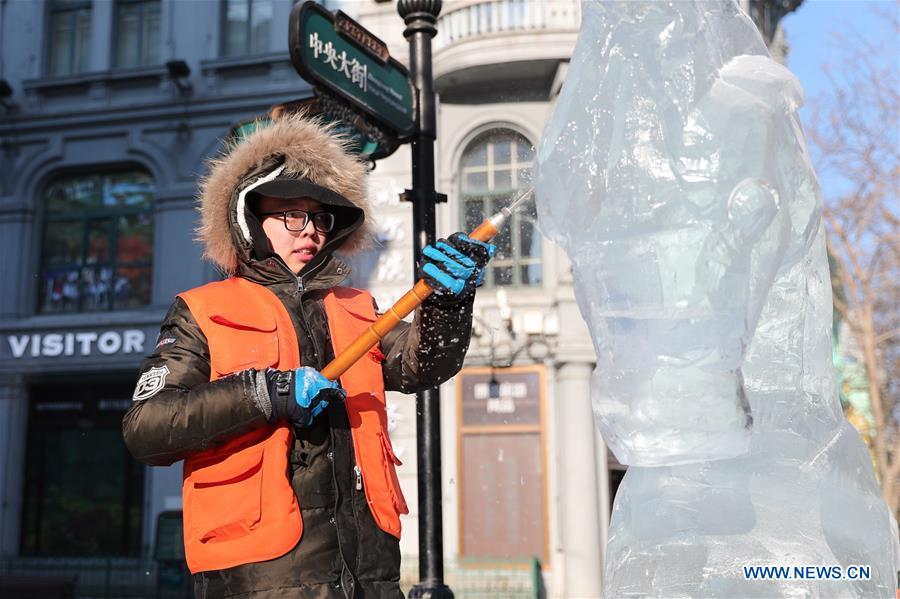In this detailed photograph, an individual is seen meticulously carving an ice sculpture of a horse on a city street. The person, who appears to be of Asian descent, is geared up with a fluorescent orange safety vest that features pockets on the front. Beneath the vest, they're wearing a dark brown jacket with a fluffy brown hood. They are also equipped with blue and black gloves and black glasses. The individual is holding an orange tool, possibly a chisel or some kind of scraping instrument, aiming it skillfully at the ice sculpture. A black street sign with green-colored signs is visible in the background, along with a gray stone building featuring brown wooden doors and a sign that reads "Visitor." The bottom of the photo notably includes the text "www.news.cn," hinting that this might be a still from a news segment. Some street signs in an Asian script solidify the urban and possibly East Asian locale of the scene.